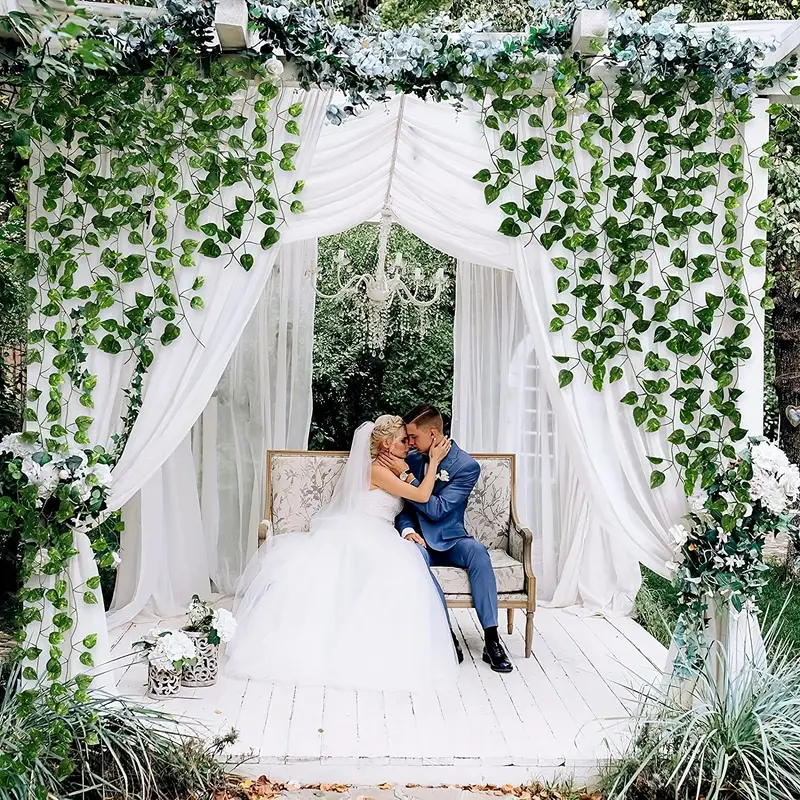In this captivating wedding photo, the newlywed couple sits intimately on a floral settee adorned with beige cushions, within a charming gazebo draped in flowing white fabric. The bride, radiant in a traditional long white wedding dress, and the groom, dapper in a modern blue suit with black shoes, touch foreheads tenderly as they hold each other close, lovingly gazing into each other’s eyes. Surrounding them, lush English ivy and white flowers complement the serene outdoor garden setting, with verdant trees visible in the background. Above them, a white chandelier adds a touch of elegance, while vases filled with matching greenery and flowers enhance the romantic atmosphere. The wooden platform beneath them completes this tranquil, picturesque scene.